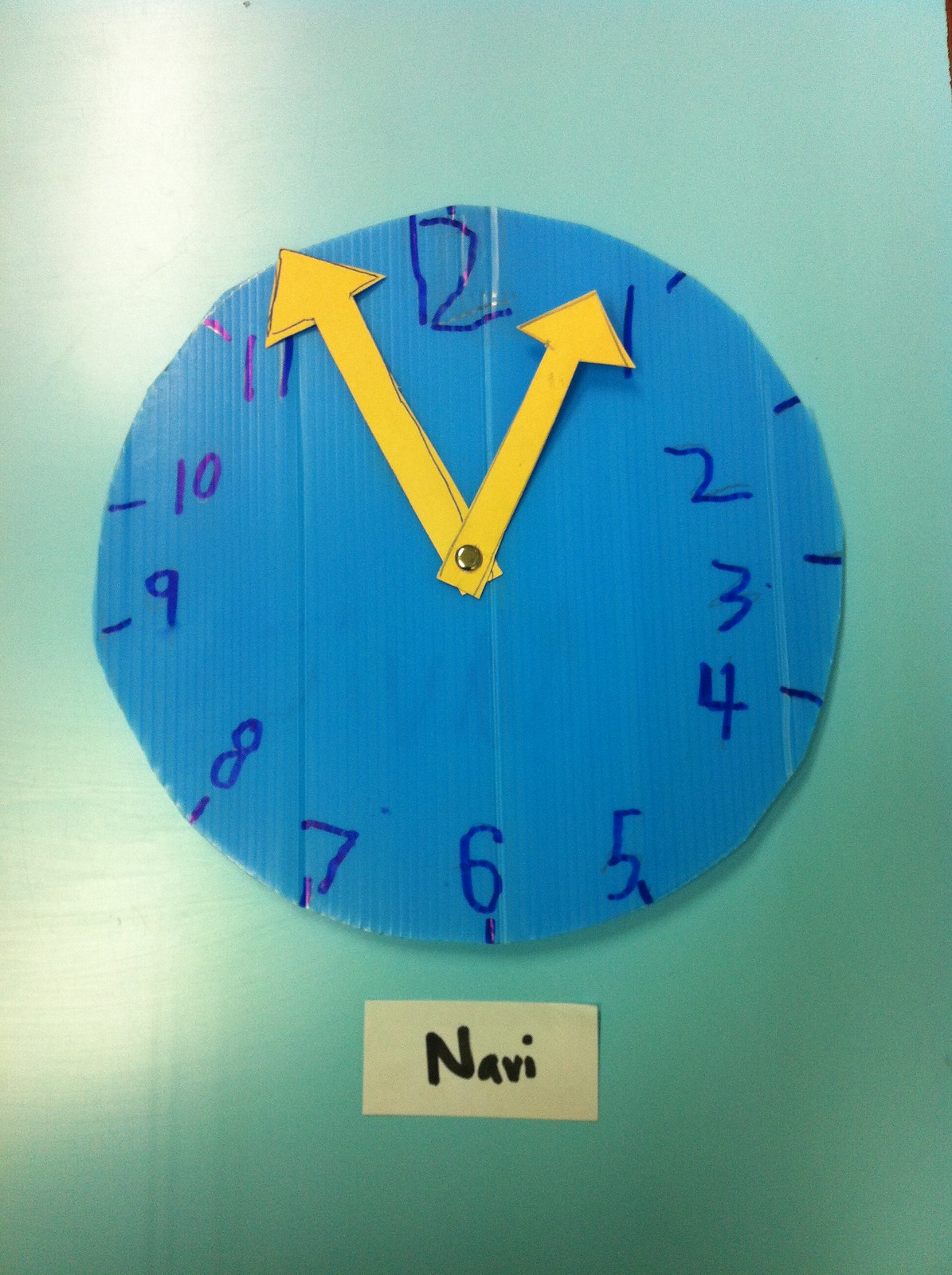This is a detailed color photograph featuring a child's handmade clock against an aqua-colored wall. The clock's face, made from a large piece of corrugated blue material, likely plastic, is cut into a rough circle with uneven edges. Blue magic marker outlines the numbers 1 through 12 in a haphazard, childlike fashion around the face of the clock. The clock hands, crafted from yellow paper and cut into arrow shapes, are fixed at the center with a tack and point between 11 and 1. Some visible pencil outlines suggest these hands were drawn and then cut out. Beneath the clock, a yellow sticky note bears the name "Navi" in black Sharpie marker. The scenario appears to capture a learning environment, possibly a teaching aid for telling time. The aqua wall's left side reflects some lighting, adding a bit of depth to the image.